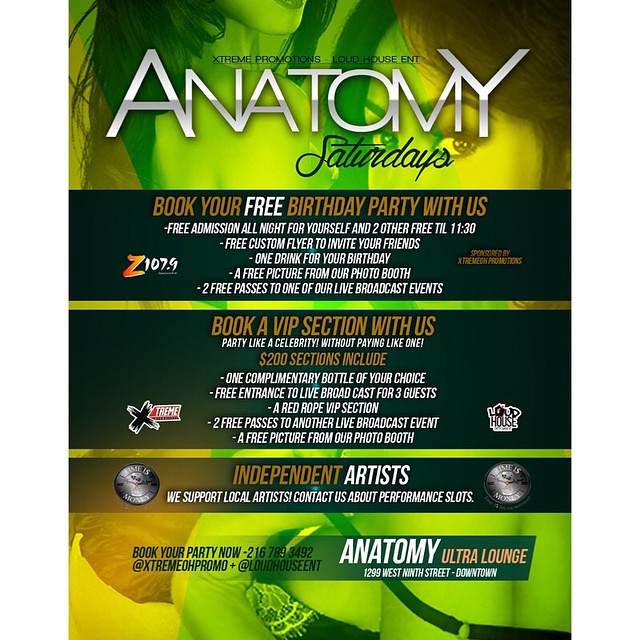Promotional flyer for "Anatomy Saturdays," presented by Extreme Promotions and Loud House ENT:

At the top, the flyer prominently displays "Anatomy Saturdays" with a cursive font for "Saturdays." Below, several black bars divide the information into sections. The first section invites you to book your free birthday party with enticing offers: free admission for you and two guests all night until 11:30 PM, a custom flyer to invite friends, one complimentary drink for your birthday, a free photo from their photo booth, and two free passes to a live broadcast event.

The second section promotes their VIP experience: "Party like a celebrity without paying like one." For $200, you can book a VIP section that includes one complimentary bottle of your choice, free entrance to the live broadcast for three guests, a red rope VIP section, two additional free passes to another live broadcast event, and a free photo from their photo booth.

The final section highlights their support for local artists. They encourage independent artists to contact them for performance slots, providing a platform to showcase their talent.

The flyer also mentions the venue's location at 1299 West 9th Street Downtown, and provides a contact number, 216-789-3492, to book your party. The backdrop features scantily clad women in club attire with a green and yellow overlay, adding to the vibrant and immersive club atmosphere.